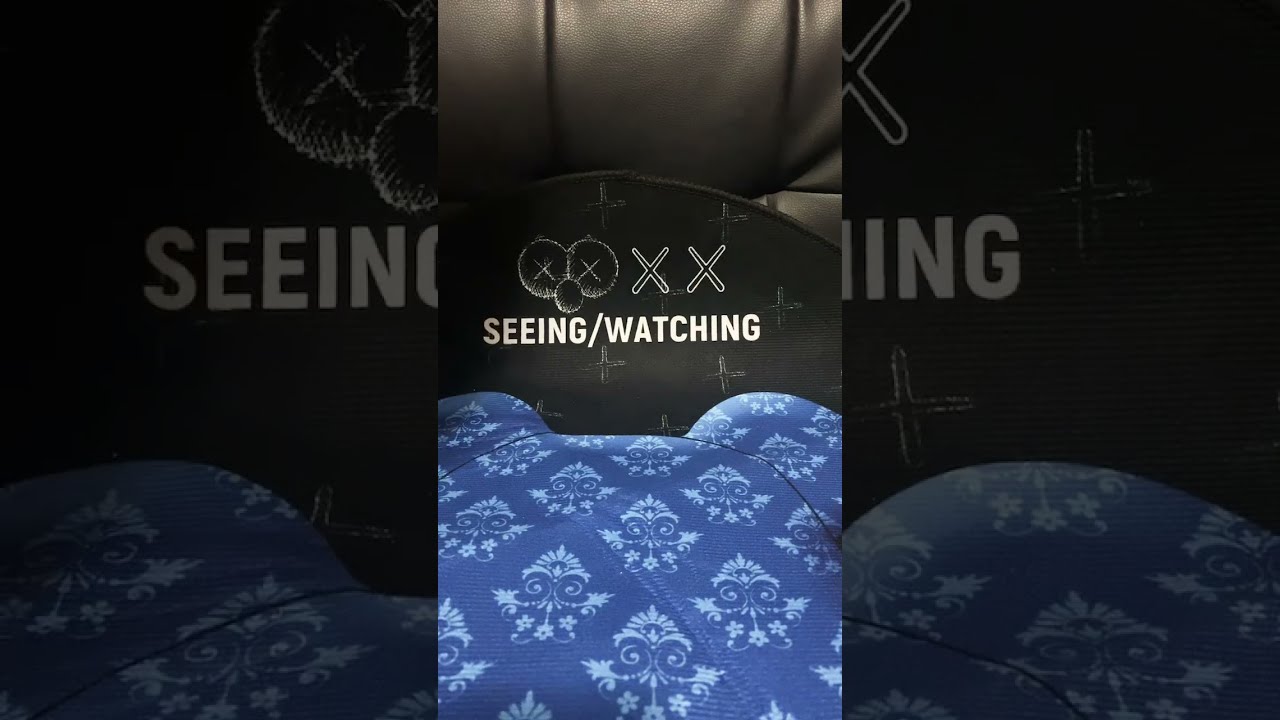The image is a detailed advertisement featuring a central panel flanked by two close-up renderings of the same panel on the left and right. The middle panel prominently showcases the words "SEEING / WATCHING" in bold, white, uppercase font against a black backdrop. Positioned above the text is a logo with four X’s: two are plain, and two are encircled, creating a face-like semblance with the circles resembling eyes and a smaller circle below hinting at a nose.

The central backdrop appears to be an arc made of black metal with intricate crosses, and in the foreground, there's a piece of blue fabric upholstery with a paisley or scroll pattern. The fabric design includes triangular shapes repeated diagonally, evocative of a richly textured pillow or cushion. The background of this central image mimics a vinyl or leather headboard with tufted stitching, enhancing the luxurious feel of the piece.

The left and right panels offer magnified views of the central scene, providing greater detail on the textures and patterns. Overall, the composition presents a sophisticated blend of text and fabric, emphasizing a sense of elegance and attentive observation.